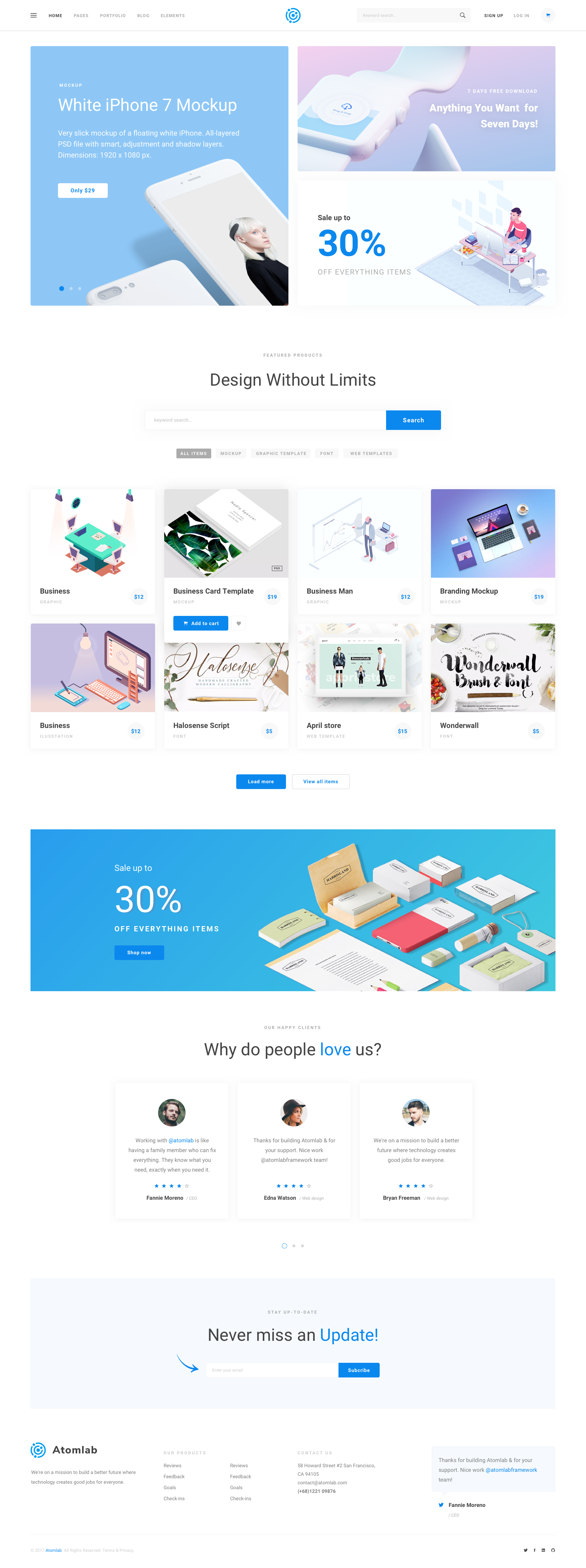The image features a horizontal menu bar located in the upper left-hand corner, which appears tiny and challenging to read. Centrally aligned on this bar is a circular logo, tinged with a bluish hue. Below the menu bar, the scene is divided into two primary sections: an image on the left and a couple of images arranged on the right.

The left section prominently displays a white iPhone 7 mock-up against a blue background. The mock-up features both the front and back views of the smartphone, with the device emerging from the bottom right corner of the image.

In the right section, there are two images stacked vertically. The top image seems to show a cable, accompanied by the text "Anything you want for seven days." Beneath it, an announcement reads "Sale up to 30%." The second image displays a person seated at a desk, with the accompanying caption "Design without limits."

Overall, the design is cohesive, integrating product mock-ups, promotional offers, and an emphasis on flexibility and creativity.